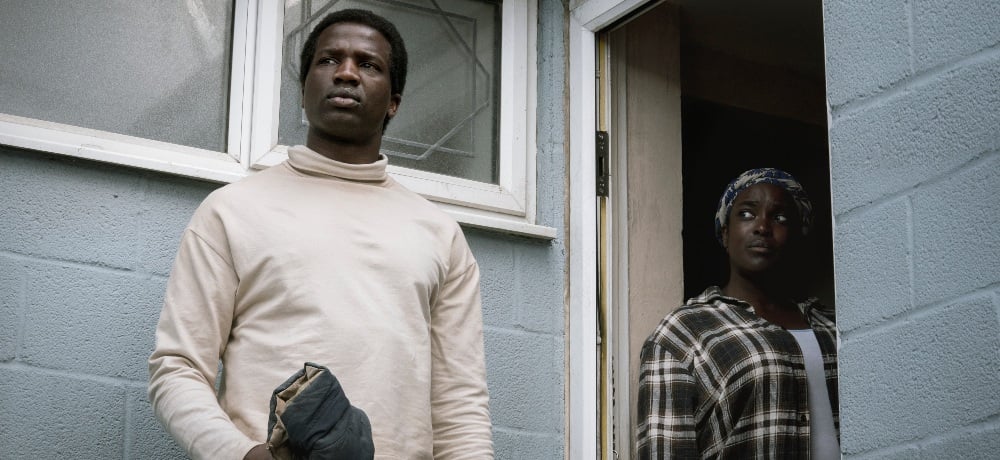In this scene, captured from what appears to be a movie or TV show, a young black man and woman stand outside a white concrete block house. The man, dressed in a cream-colored turtleneck and holding a folded gray jacket, is positioned to the left of the doorway, gazing to his left with a seemingly concerned expression. Behind him, a window with two panes and white trim is visible. The woman, likely his mother, stands in the doorway wearing a blue and white headscarf and a black and cream plaid shirt over a white blouse. She looks towards the man with a worried look, her stature shorter in comparison, suggesting she might be around 5'4" while he stands over six feet tall. The scene is framed with natural wood doors and the house’s white exterior, emphasizing the emotional distance and concern between the two characters.